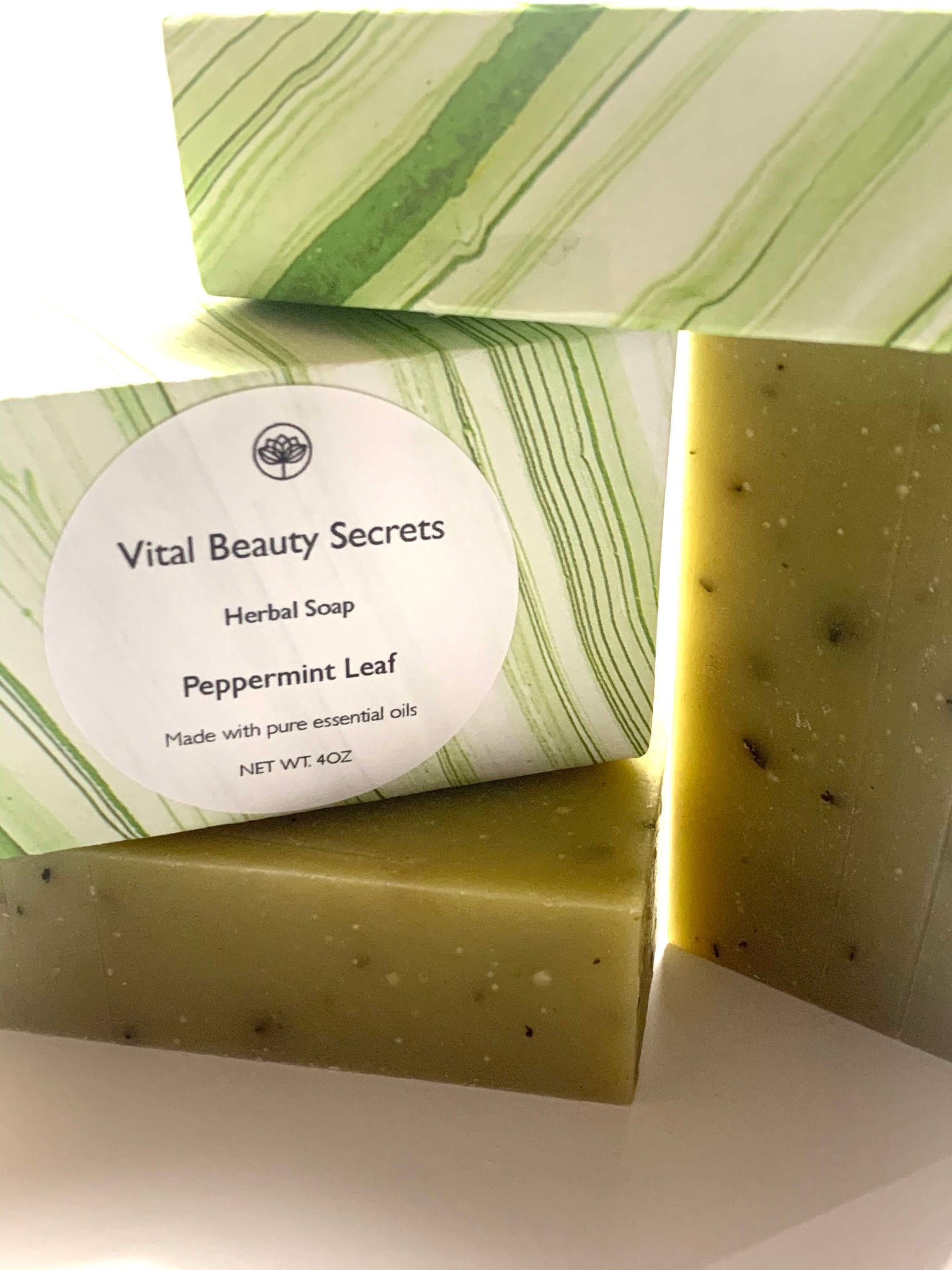The image depicts several bars of Vital Beauty Secrets Herbal Soap, specifically the Peppermint Leaf variety made with pure essential oils. The soaps are displayed on a light brown countertop with a white background. Two bars are unwrapped, revealing a murky, grassy green color speckled with black and white particulate matter, likely plant-based exfoliants. One unwrapped bar lies flat, while the other stands vertically. Beside them, two wrapped bars rest on top of the unwrapped ones. The wrappers feature a green and white swirly stripe pattern, angled from the upper left corner to the bottom right, with a circular label containing the brand name, product type, and details about the soap in black text. The detailed packaging adds an artisanal touch, suggesting this could be an item featured on Etsy or Instagram. The net weight of each soap is 4 ounces. Bright light illuminates the scene, highlighting the texture and appearance of both the soap bars and their packaging.